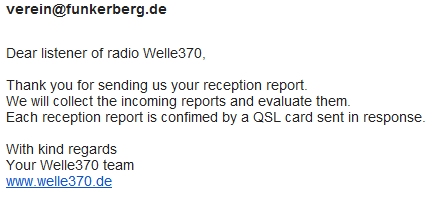The image displays an email correspondence on a white background. At the top, in bold black font, is the email address "verein@funkerberg.de". The body of the email reads: "Dear listener of Radio Welle 370 (spelled W-E-L-L-E 370), thank you for sending us your reception report. We will collect the incoming reports and evaluate them. Each reception report is confirmed by a QSL card sent in response. With kind regards, your Welle 370 team." Below the closing, there is a hyperlinked address "www.welle370.de" in blue. The text is formatted in Arial font, and the layout suggests it is a standard email, despite lacking a subject line.